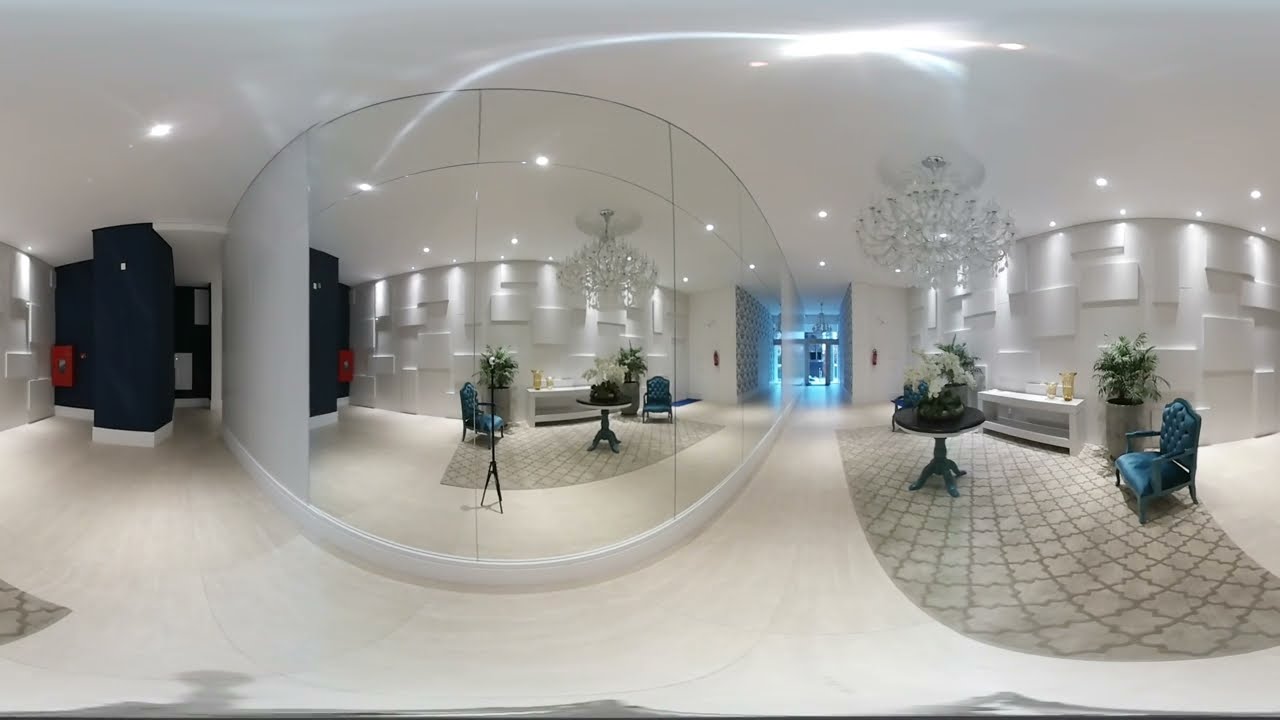This photo, taken indoors with a fisheye lens that distorts the perspective, features a spacious and immaculately clean lobby, which could belong to a hotel, an apartment building, or an office. Dominated by a giant wall mirror on the left side, the room is well-lit with numerous lights and a large crystal chandelier hanging prominently from the ceiling. The floor is spotless and white, with a unique curvature due to the lens effect. This elegant space includes a royal blue velvet chair positioned near a green plant and small wooden tables adorned with flowers and decorations. In the background, there's a visible walkway leading to a blue-lit area, and safety equipment like a fire alarm and an extinguisher is also present. Despite the luxurious and welcoming arrangement with cozy seating and refined décor, there is nobody around, emphasizing the serene and undisturbed atmosphere of this lobby.